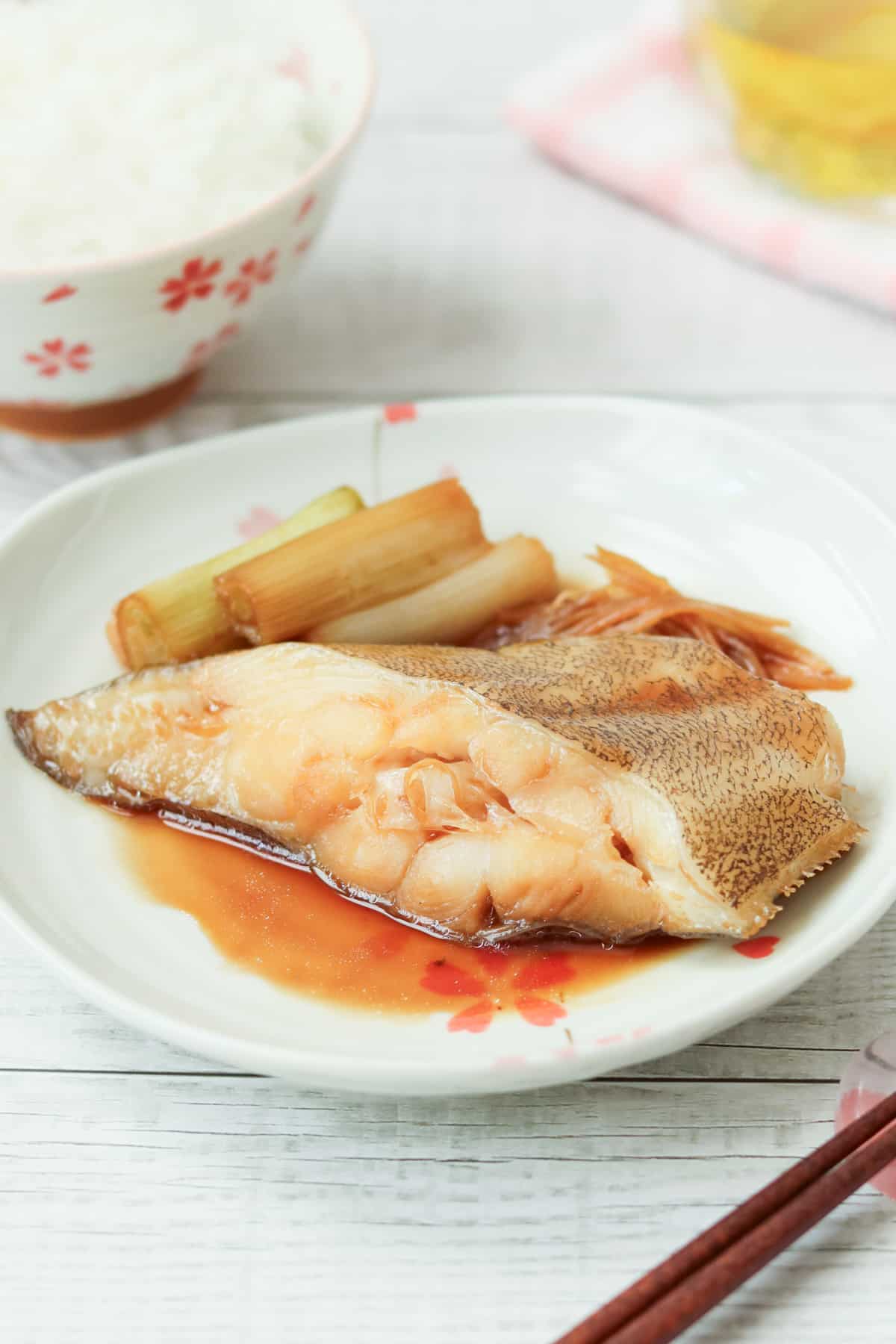This photograph captures an intricately arranged dish of fish, likely sashimi, displayed on a white plate adorned with pale pink flowers. The angling of the fish reveals its tender, white meat and a visible center bone, suggesting it's uncooked. The surface of the fish is characterized by an orangish-white hue with black stripes forming a gridlock pattern. A rich orange sauce, possibly soy-based, seeps out from underneath the fish, creating an alluring contrast against the plate. Surrounding the fish are three unique, pale green vegetables tinged with orange, resembling larger green onions or leeks, indicating they might be cooked or pickled. Adjacent to the fish, a stringy, orange food item adds another layer of texture to the arrangement. The dish is part of a larger setting atop a white-stained wooden table. In the blurred background, a pink and white plate holds a yellow dish, while a white bowl with pink flower patterns filled with white rice is visible. On the very bottom right edge of the frame, partially cropped, is a pair of chopsticks placed across another pink and white dish.